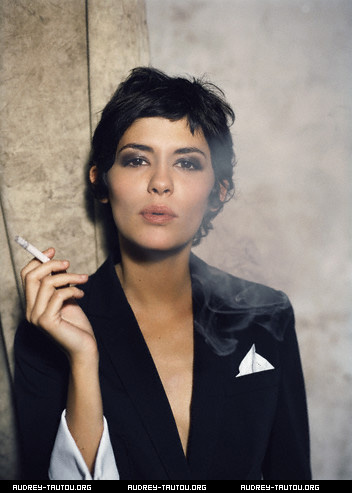The image features a young woman with short black hair, standing confidently against a backdrop that appears to be a white curtain wall or possibly a wooden background. She is wearing a black blazer with white cuffs and a pocket square prominently displayed in the front pocket, seemingly without a shirt underneath, revealing her skin. She is pictured from the waist up, holding a lit cigarette in her right hand, which is pressed against her body, and she is blowing smoke towards the camera. Her makeup is striking, with heavy eye makeup including black eyeshadow and eyeliner, well-defined eyebrows, and slightly pink lips. She looks directly into the camera, adding a sense of intensity to the shot. The bottom of the image displays "AudreyTatou.org" repeated three times.